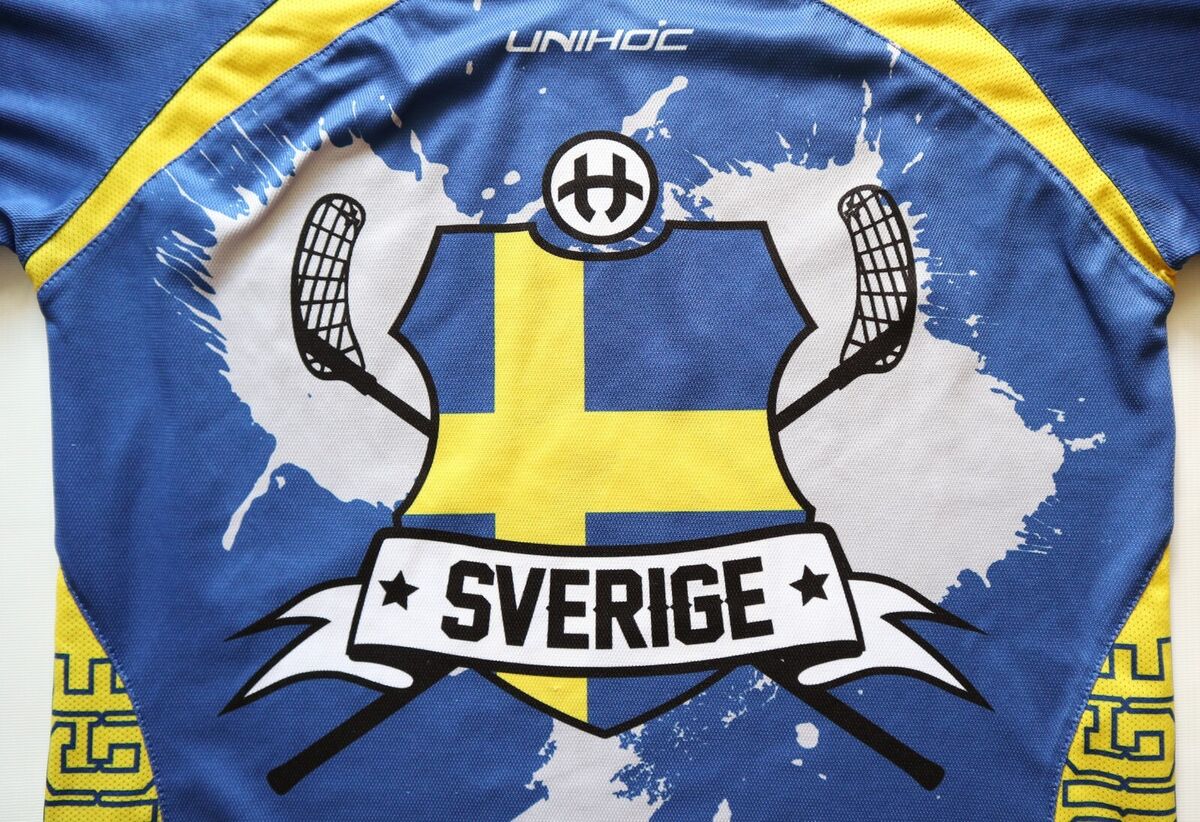The image appears to be a sports jersey, possibly for field hockey, showcasing a blue and yellow color scheme with white accents. The main design includes a central shield-like crest featuring a yellow cross on a blue background. Above the crest, it reads "UNI HOC" with a distinctive circular logo containing an ornate "H." Below the crest, a banner with the word "SVERIGE" in black text is flanked by two black stars. The background includes a white paint splatter effect and what looks like field hockey sticks, enhancing the sporty appearance. The country indicated by "SVERIGE" is likely Sweden.